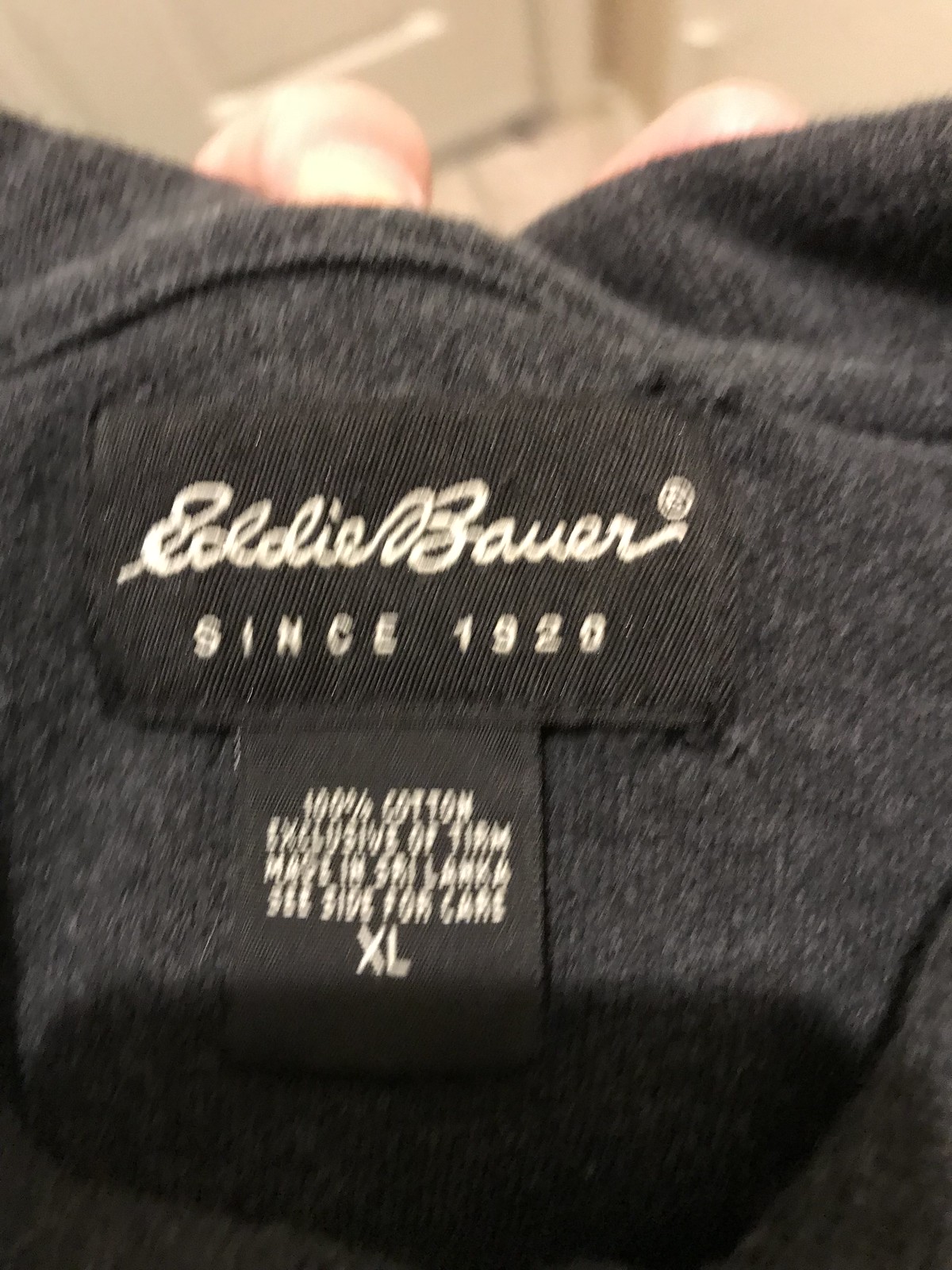The image captures a slightly blurry close-up of a clothing tag attached to a charcoal gray garment with a lightly fuzzy, fleecy texture. The black tag features "Eddie Bauer" written in cursive white text, followed by "Since 1920" printed underneath. Below this, a smaller, squarish tag states "100% cotton, exclusive of trim," and "Made in Sri Lanka," along with washing instructions and the size "XL." Additionally, the image includes the fingers of the person holding the shirt, specifically, an index finger and part of a middle finger, which are visibly Caucasian.